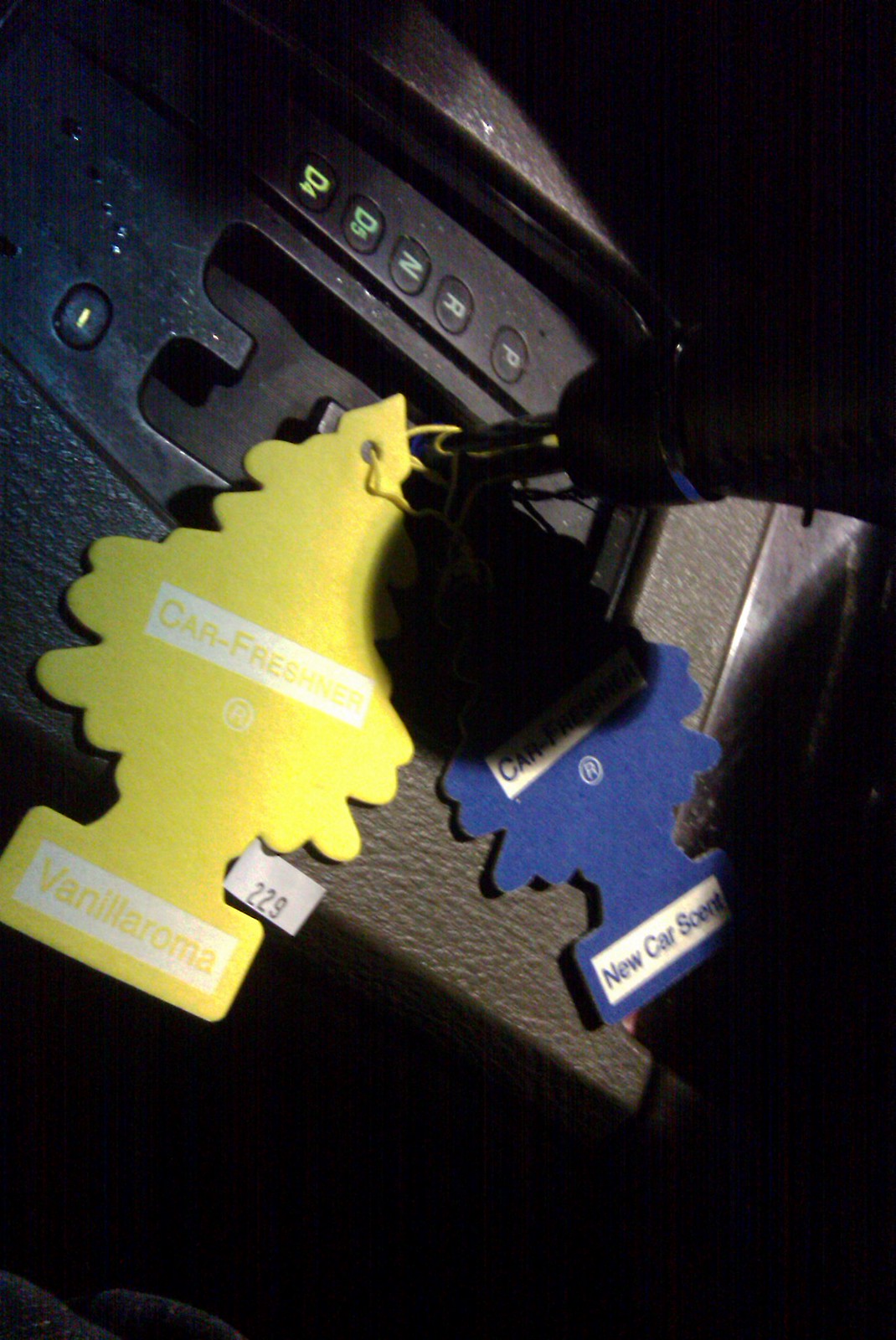The photograph, which appears to be taken from the passenger seat of an American vehicle, showcases the black automatic gear lever positioned currently in 'Park'. The image captures the black center console of the car, shrouded mostly in shadows likely due to low lighting conditions. The shadows create a dark background especially prominent in the top right and lower sections. Notably, two pine tree-shaped air fresheners dangle around the gear lever; one is yellow labeled "vanilla" with a price tag reading $2.29, and the other is blue labeled "New Car Scent". Additionally, the surface of the console appears to have small drops of water, indicating possible condensation or spillage. The gear letters, 'P', 'R', 'N', 'D', 'D4', and 'D5' are clearly visible in white text, aligning to the left of the gear shifter.